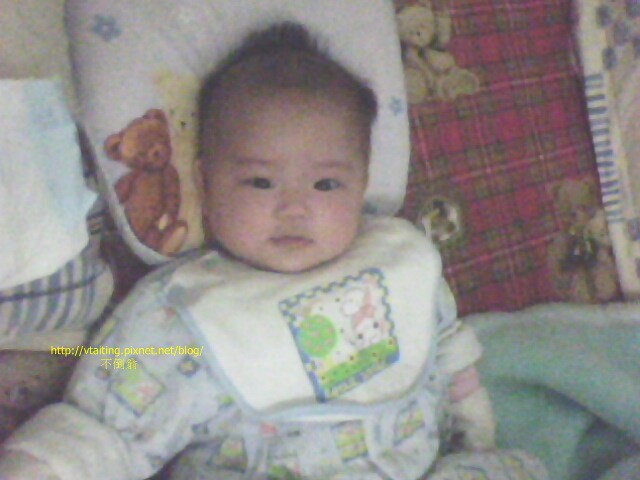This faded, full-color photograph captures an adorable young Asian baby, likely a girl, resting on a white pillow adorned with flower designs and two teddy bear prints. The baby, clad in a white bib decorated with a bear and possibly a tree, also wears tiny mittens to prevent self-scratching. She lies on a plaid-patterned surface in hues of red, brown, and black, which features additional teddy bears. Although the image is somewhat blurry and possibly rotated, the details evoke a tender and nostalgic glimpse into a cozy, cherished moment.